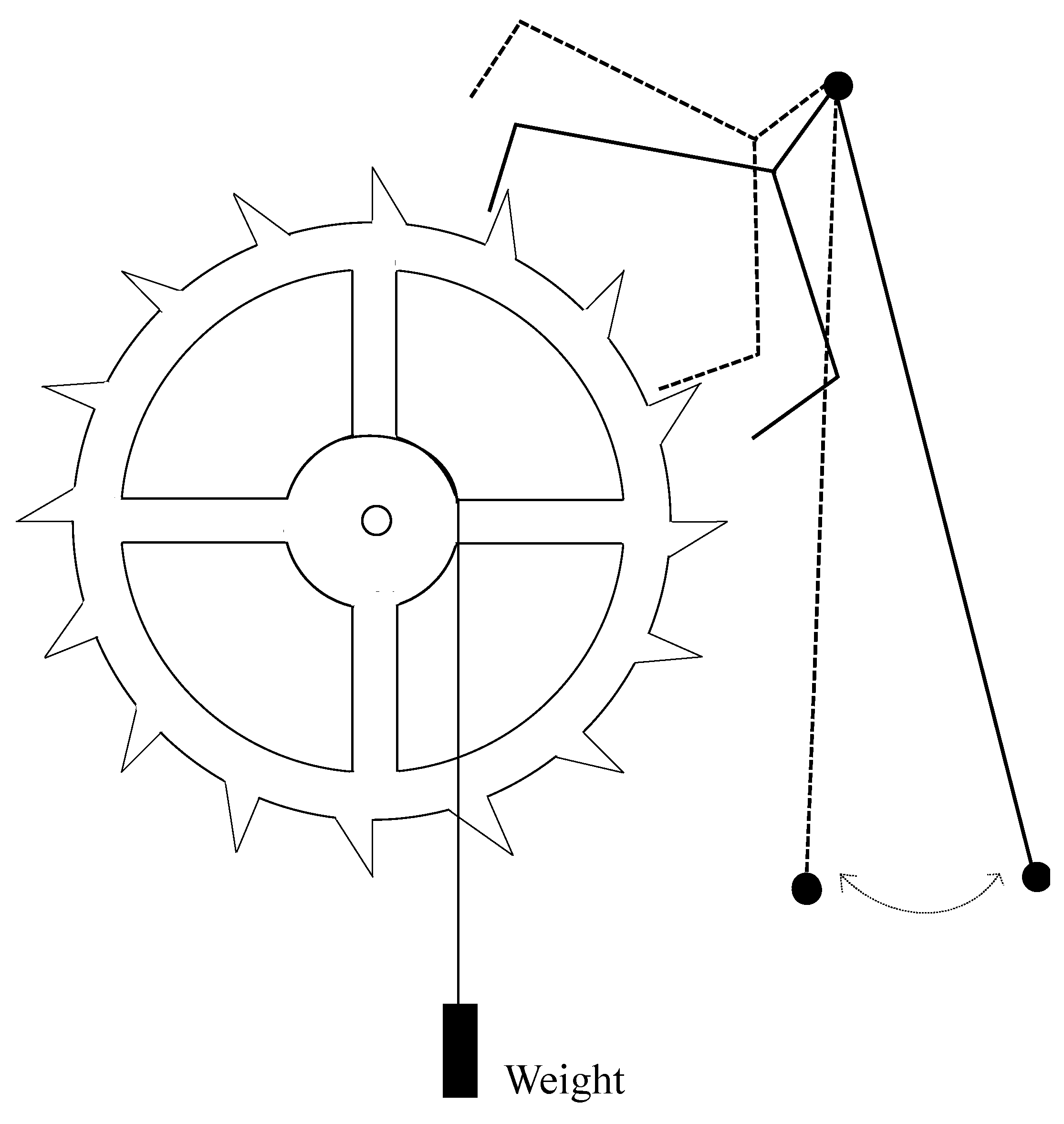In this black and white diagram, we observe a detailed depiction of a basic mechanical apparatus. At the center is a spoked wheel segmented into four parts, encircled with sharp, spike-like edges. A string is attached to this wheel, holding a solid object labeled "weight," which is crucial in the operation depicted. As the wheel turns, these spikes engage with a metal structure on the right, triggering a motion that causes long, weighted wires, likely strings, to swing back and forth in a rhythmic pattern. Additionally, there is another structure of arms adjacent to the wheel, which appears to aid in propelling the wheel’s movement. This simple yet intricate mechanism demonstrates the interplay between the spoked wheel, the sharp-edged spikes, and the swinging weighted wires, all contributing to its perpetual motion.